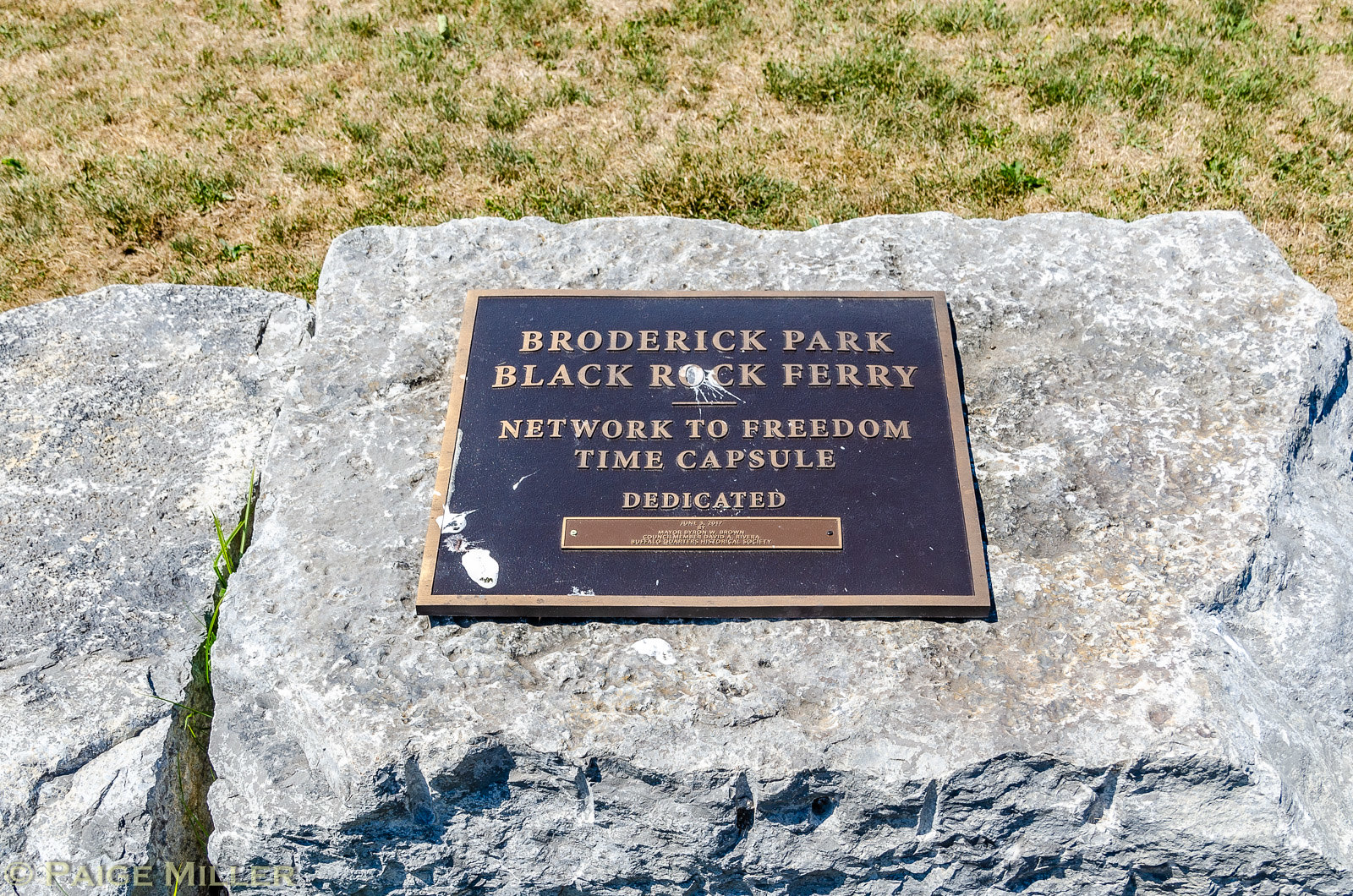The image captures an outdoor scene of a monument featuring a large, gray, rectangular rock with a black and gold plaque affixed to its surface. The plaque, which appears to have raised copper lettering, bears the inscription: "Broderick Park, Black Rock Ferry, Network to Freedom, Time Capsule, Dedicated." Below this main inscription is a smaller, unreadable rectangular segment, likely additional information about the monument. The rock shows signs of bird droppings in various spots. Adjacent to this rock is a smaller, similar gray rock. The surrounding environment consists of a grass field that appears to be deteriorating, with patches of green interspersed with areas of faded, beige grass. The scene is bathed in daylight, indicating that the photo was taken during the day. In the gaps between the rocks, grass and weeds can be seen growing.